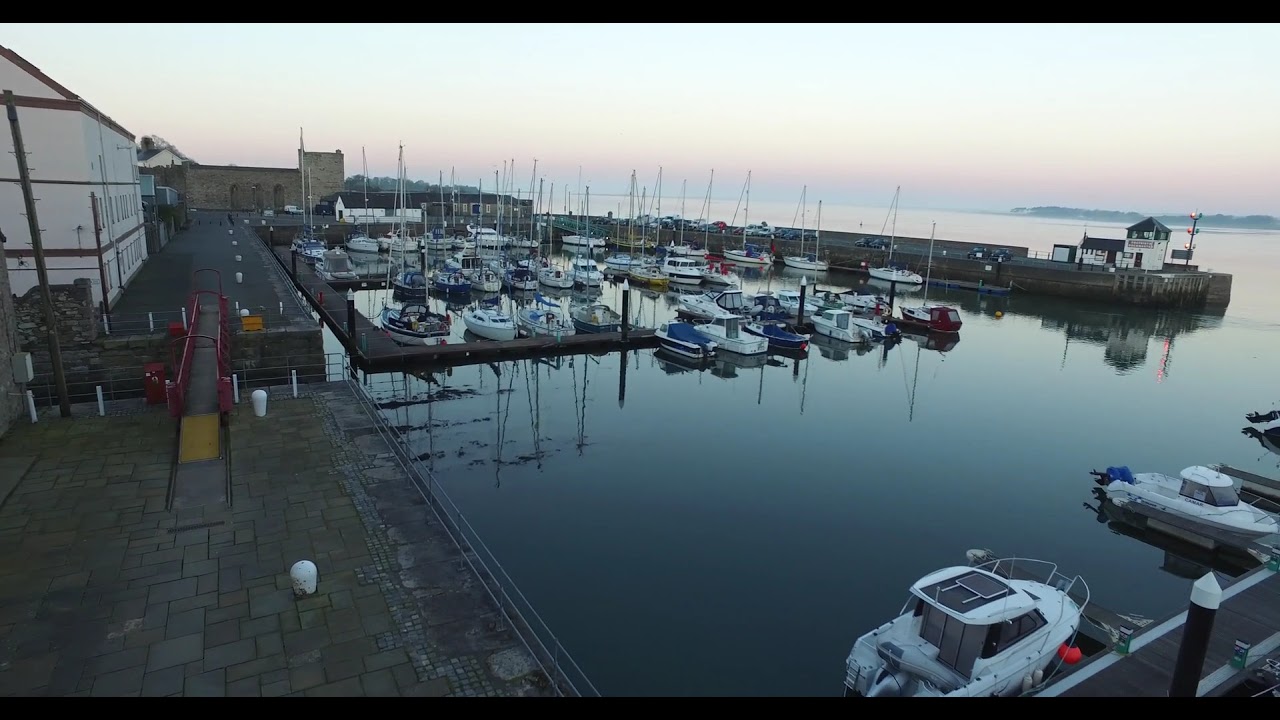The image is a horizontally aligned rectangular shot, taken from a high-angle viewpoint, possibly from a building, roof, or parking garage, overlooking a serene harbor. The scene captures the early morning light, painting the sky a light blue with hints of pink. The water below is mostly calm, with no visible ripples, stretching off to the distant horizon, which could be an ocean or a large lake.

In the foreground below the vantage point, there is a concrete or brick-paved area that extends directly to the water's edge. Numerous wooden piers stretch out into the harbor, creating multiple docking spaces filled predominantly with sailboats, identifiable by their masts, and smaller personal craft. The boats are lined up neatly with floating walkways in between.

On the left side of the image stands a prominent three-story white wooden building with a house-like roof, appearing more like a facility related to the marina. Adjacent to this building is a stone walkway with a metal barrier, and a notable red footbridge crossing one of the waterways.

Towards the upper part of the image, a stone port area with a lighting tower, possibly serving as the Harbour Master's outlook, is visible on the right. The background features outlines of hills or trees with a light blue sky above, adding depth to the serene morning harbor scene.